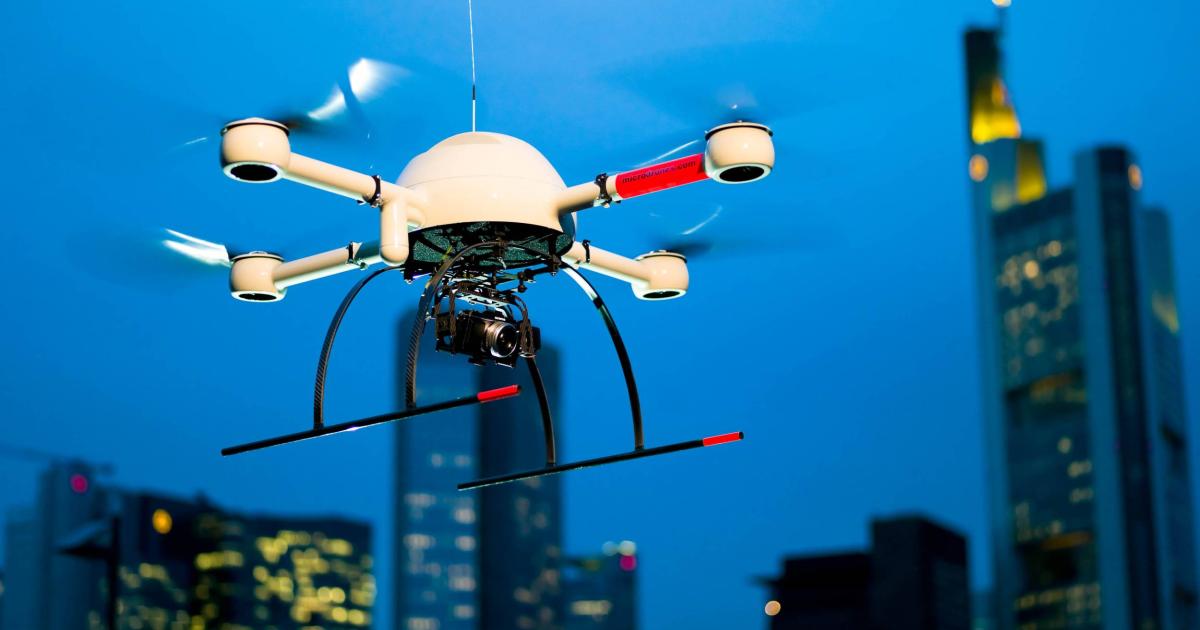In the dim, twilight sky of a bustling city, a white drone hovers prominently in the foreground, framed by a backdrop of towering skyscrapers. The sky is dark blue, hinting that night has just fallen and the sun has recently set. The buildings behind it are bathed in various shades of blue, with many windows illuminated, casting a glow against the darkening firmament. The drone features a hemispherical shape with four white arms extending outward at right angles, each equipped with a rotor blade. Beneath the drone, a small, camera is mounted, resembling a miniature Canon camera. Supporting the drone are black metal landing skids with red-tipped ends, shaped like C's welded together at the bottom, enabling it to touch down safely. Together, these elements capture a sleek, modern simultaneity between the urban landscape and advanced technology.